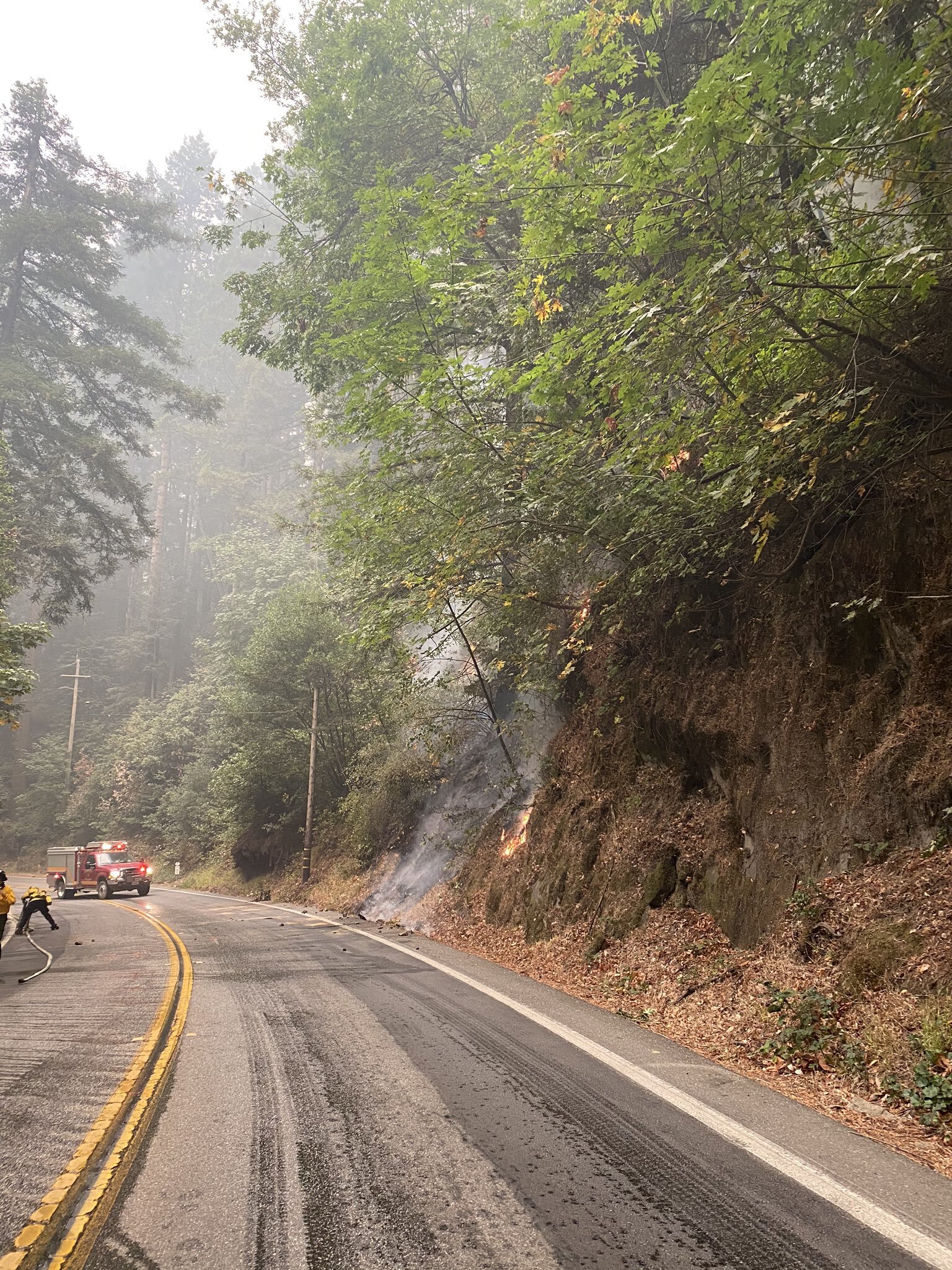In this photograph, a firetruck is stationed on a curved, two-lane road in a densely wooded, rural area, surrounded by vibrant green trees. On the left side of the image, two firemen are working with a hose, aiming to control the situation. To the right of the road, which features two yellow lines indicating a curved section, there is a steep, rocky bank with trees growing out of it. A small fire has ignited in the brush alongside this cliff, with visible orange flames and smoke rising from both the bottom and higher up, creating a smoky haze. Water is evident on the road, suggesting ongoing efforts to extinguish the flames. The firetruck is positioned in the middle of the road, close to a corner, highlighting the urgency and active response to the burgeoning fire hazard.